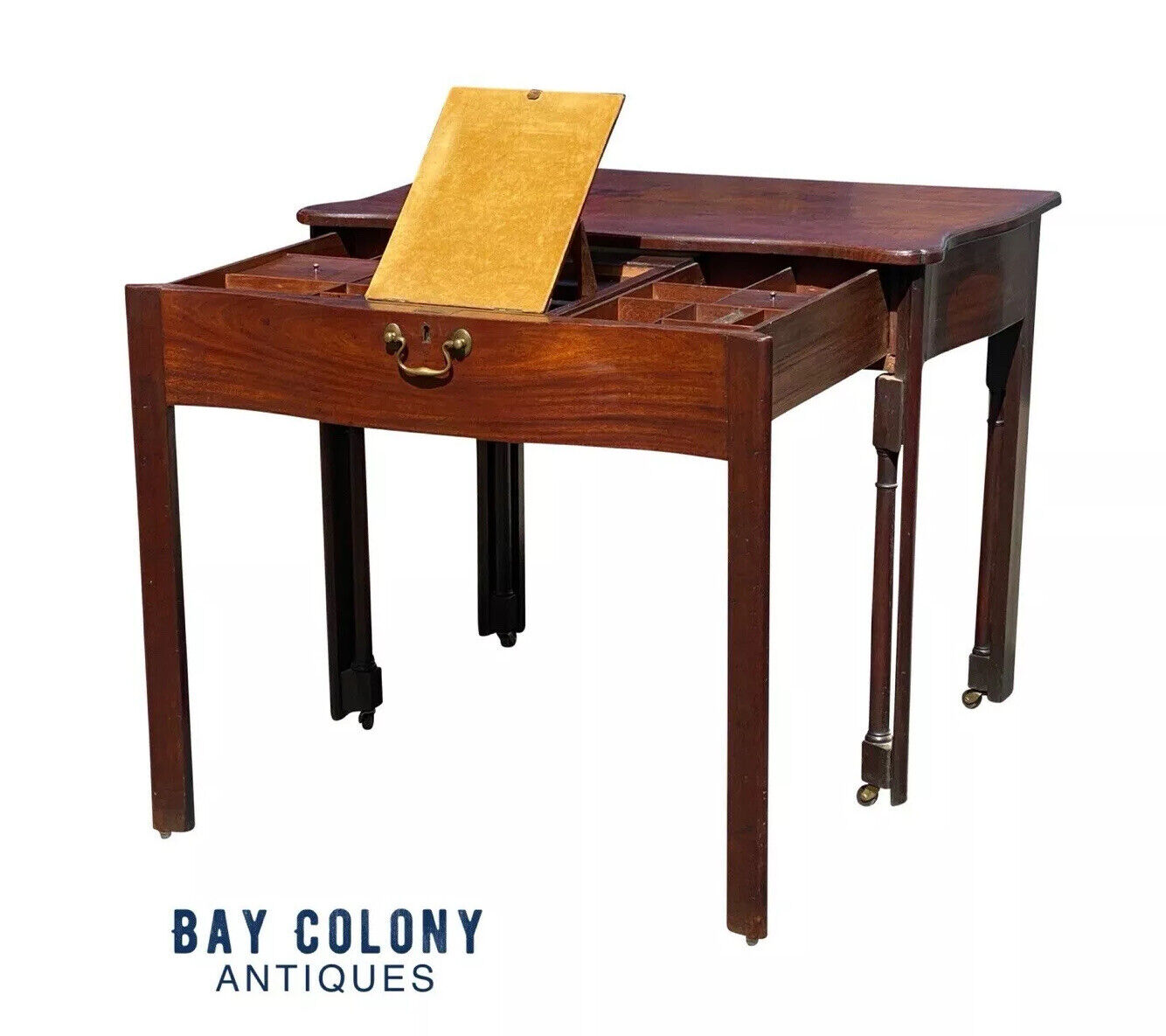The image presents a vertical, antique drawing table made of reddish-brown wood, prominently displayed by Bay Colony Antiques as indicated by the black letters in the lower left corner. The elegant table features four main legs, each equipped with wheels for easy mobility. A distinctive element is its large drawer, which can be pulled out and reveals numerous partitions inside. The drawer is supported by an additional leg, making the table appear to have six legs when extended. This extra leg cleverly fits inside the table's front legs when the drawer is closed, maintaining a seamless four-legged appearance. The drawer is adorned with a bronze pull handle. On top of the drawer sits a light brown, rectangular board, and inside, there's a manila envelope propped up, likely indicating the table's use or an additional feature. This intricately designed piece encapsulates both functionality and historic charm.